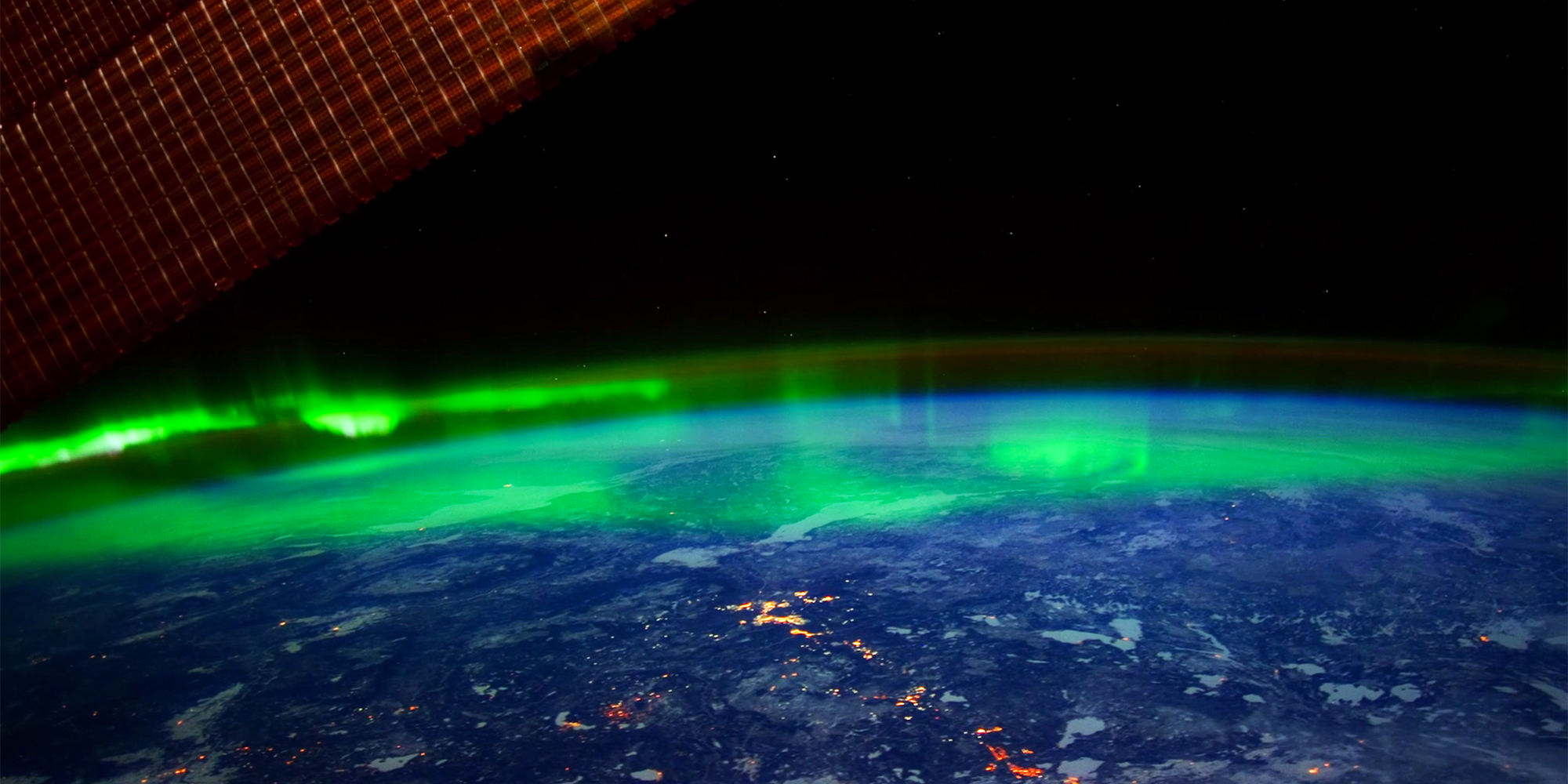The image depicts a full-color view of Earth from space, framed horizontally without a border. The backdrop is the black void of space, devoid of stars or text. Dominating the scene is the vivid green arc of the aurora borealis, which stretches slightly curved across the middle, becoming especially bright towards the center left. Earth's surface, visible beneath the aurora, appears as indistinct patches of land and water, interspersed with heavily lit-up areas in yellow and red, likely infrared representations of city lights. The overall surface tone transitions between shades of blue, indicative of both land and water, though specific continents are indistinguishable. In the upper left corner, a section of a satellite, potentially an orangish solar panel, is visible, adding to the context of the image being captured from space.